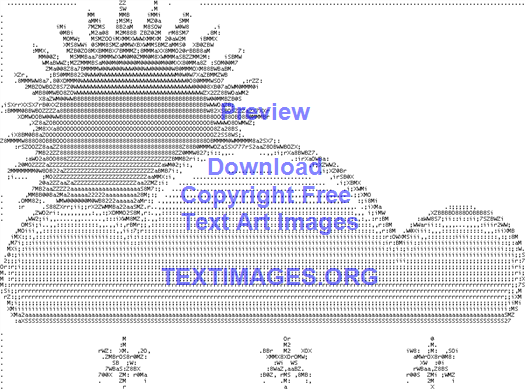The image depicts a piece of ASCII text art set against a white background, ensuring the black characters stand out sharply. In the upper left, a detailed sun with numerous pointed rays emerges, casting its light onto a cloud formation below. The cloud comprises three main circular humps with the largest circle centrally positioned. Beneath this cloud are three star-like or snowflake-shaped figures. Across the image, there’s blue text stating, "Preview, download copyright-free text art images," followed by "textimages.org." The overall design is pixelated, suggesting a digital or computer screen origin, with clear emphasis on the intricate patterns created by the ASCII characters.